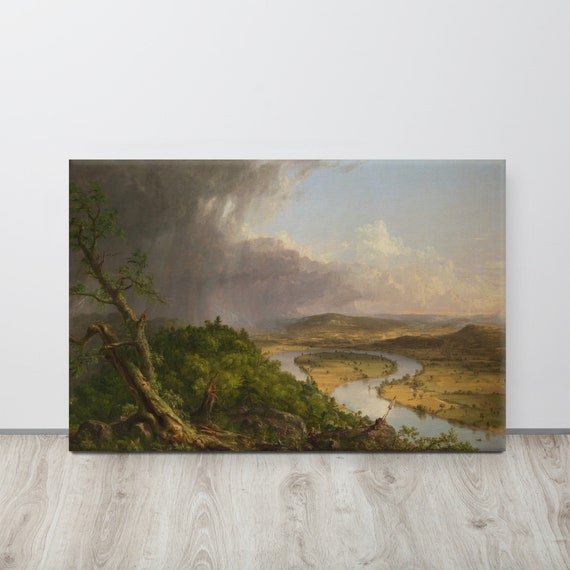The image depicts an unframed painting leaning against a white wall on a light-colored wood-grained floor, likely in an art gallery. The painting features a natural scene with a river winding in a C-shape through a hilly, vegetated landscape. To the right side of the painting, the river curves around, bordered by green trees and bushes in the foreground. A partially fallen tree trunk lies on the left side, with remnants of cut branches and a few leaves. The background shows a mix of blue sky and ominous dark clouds suggesting impending weather, situated above the undulating terrain. The painting has a thick, raised surface, emphasizing its craftsmanship.